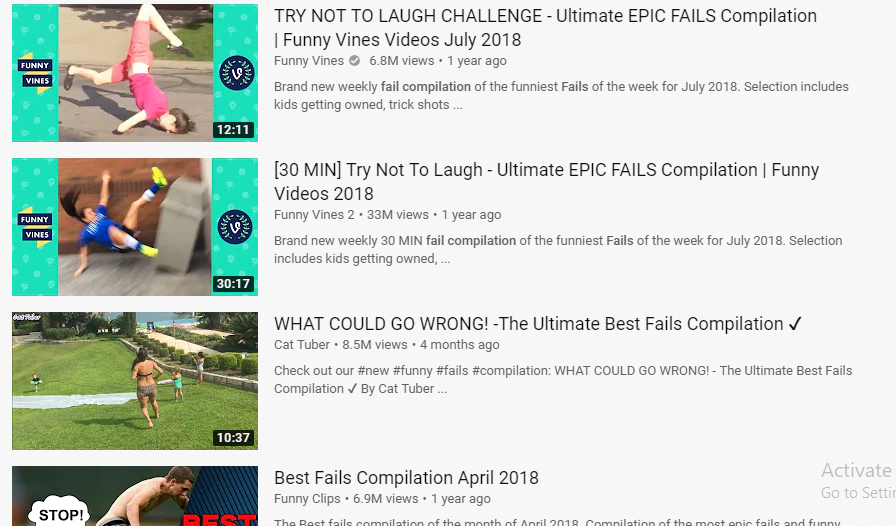Screenshot of a video app or website showcasing four video thumbnails on the left side of the screen with corresponding details to the right. The top thumbnail displays a person face-down on asphalt with their feet in the air. The title reads: "Try Not to Laugh Challenge Ultimate Epic Fails Compilation Funny Finds Videos July 2018." Below, another thumbnail features a girl falling in front of a trash can. The video details, including title, content creator, view count, and posting date, appear to the right of each thumbnail. The third thumbnail shows a woman standing on a large lawn with children, titled: "What Could Go Wrong: The Ultimate Best Fails Compilation." The bottom thumbnail is partially cut off, depicting a shirtless man with a cartoon speech bubble saying "Stop" behind him. The title is: "Best Fails Compilation April 2018."